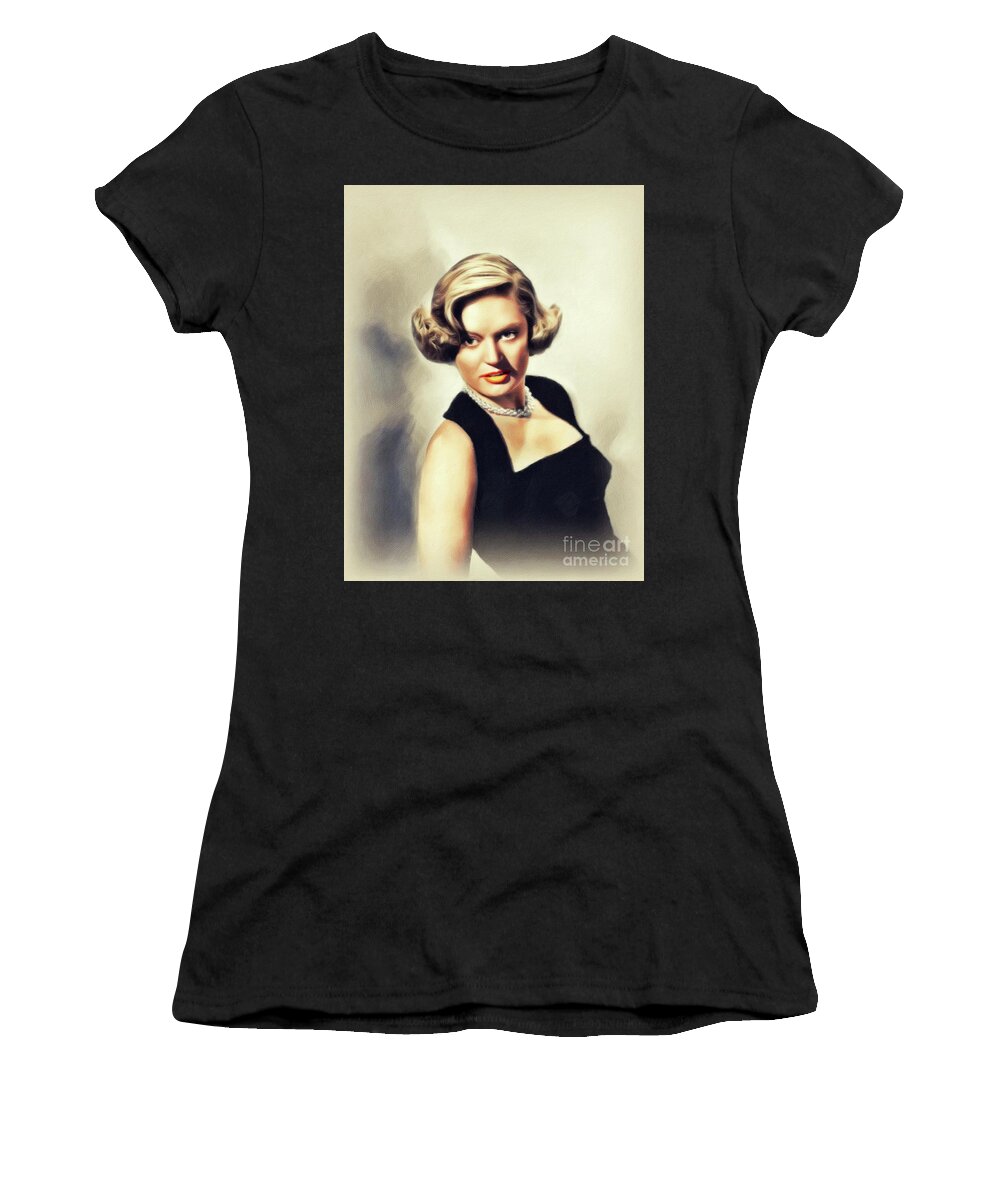This is an image of a women's black short-sleeved T-shirt, displayed against a plain white background. The shirt, made from cotton, features very short sleeves and a round collar, with a realistic depiction that includes slight wrinkles in the fabric. The focal point of the T-shirt is a vertically oriented rectangular image just below the collar, resembling a vintage photograph but rendered in a painting style. The background of the image is light gray with a darker gray on the left side. It showcases a woman with short, blonde hair styled so that it curls up at the ends. The woman, who has a seductive expression with red lipstick, is depicted wearing a black cocktail dress with straps over her shoulders and a straight neckline above her chest. She also sports a silver necklace. Her body is partially turned to the right, but her head is turned back towards the viewer. The image extends down to her midsection. At the bottom right corner of this printed image, there is faint writing that reads "Fine Art America."